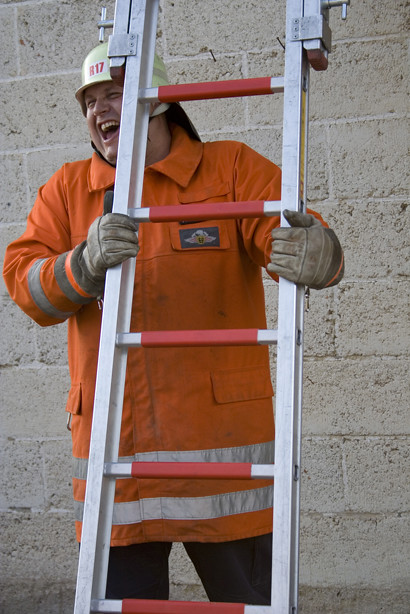This image captures a jovial, slightly heavy-set white firefighter standing behind a silver extendable ladder with red prongs. He is wearing a light greenish firefighter helmet marked with "R-17" in red, and a classic orange fireproof jacket featuring reflective silver stripes around the waist and arms. His hands, clad in heavy-duty gloves, are firmly gripping the ladder, which appears ready to be set up against the backdrop of a concrete block wall with exposed nails. The firefighter, whose face is lit up with a broad smile as he looks off to the left, seems to be enjoying a light-hearted moment, rather than hurrying to combat a fire. His blue pants complete the uniform, contributing to the overall image of a cheerful day on duty.